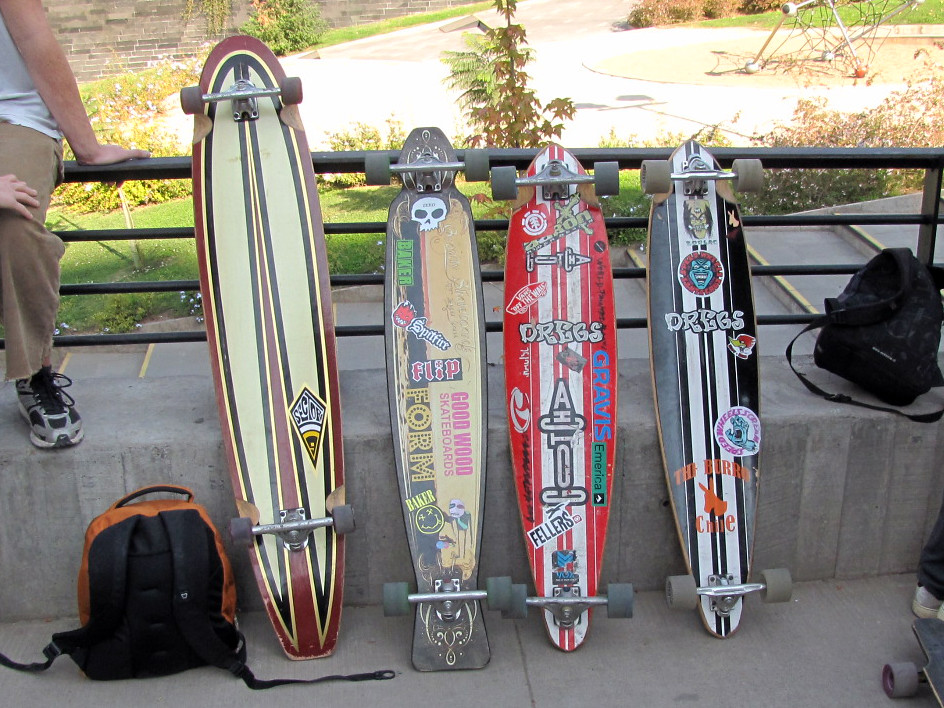This image captures an outdoor scene on a sunny day, showcasing four longboard skateboards propped against a metal railing. The background reveals a street, green lawns, bushes, and some trees. The railing sits atop a thick concrete divider positioned along a set of concrete steps with yellow accents. 

A person in brown pants, gray tennis shoes, and a white t-shirt sits on the left side of the railing, partially in frame. Their hand is grasping the back of the rail, and at their feet lies an orange and black backpack. Nearby, a black and brown skateboard with a white, elongated design rests against the divider.

From left to right, the showcased longboards are:
1. A maroon board featuring yellow and black stripes that taper to a point.
2. A primarily brown and black board with various logos and stickers, including "FORM" in yellow, "Goodwood Skateboards" in hot pink, a skull, and a caricature with red and blue eyes.
3. A red and white board adorned with various stickers and bumper stickers, including the word "DRUGS."
4. A black and white striped board, also covered in stickers and bearing "DRUGS" and a circular design with a monstrous green face, white teeth, and yellow eyes.

All four boards have gray wheels. On the right side of the image, a black backpack rests on the concrete divider, next to another skateboard whose wheels and tail are just visible. The image brims with details of the skateboards' graphics and the surrounding environment, encapsulating a casual, sunny day in a lush outdoor area.